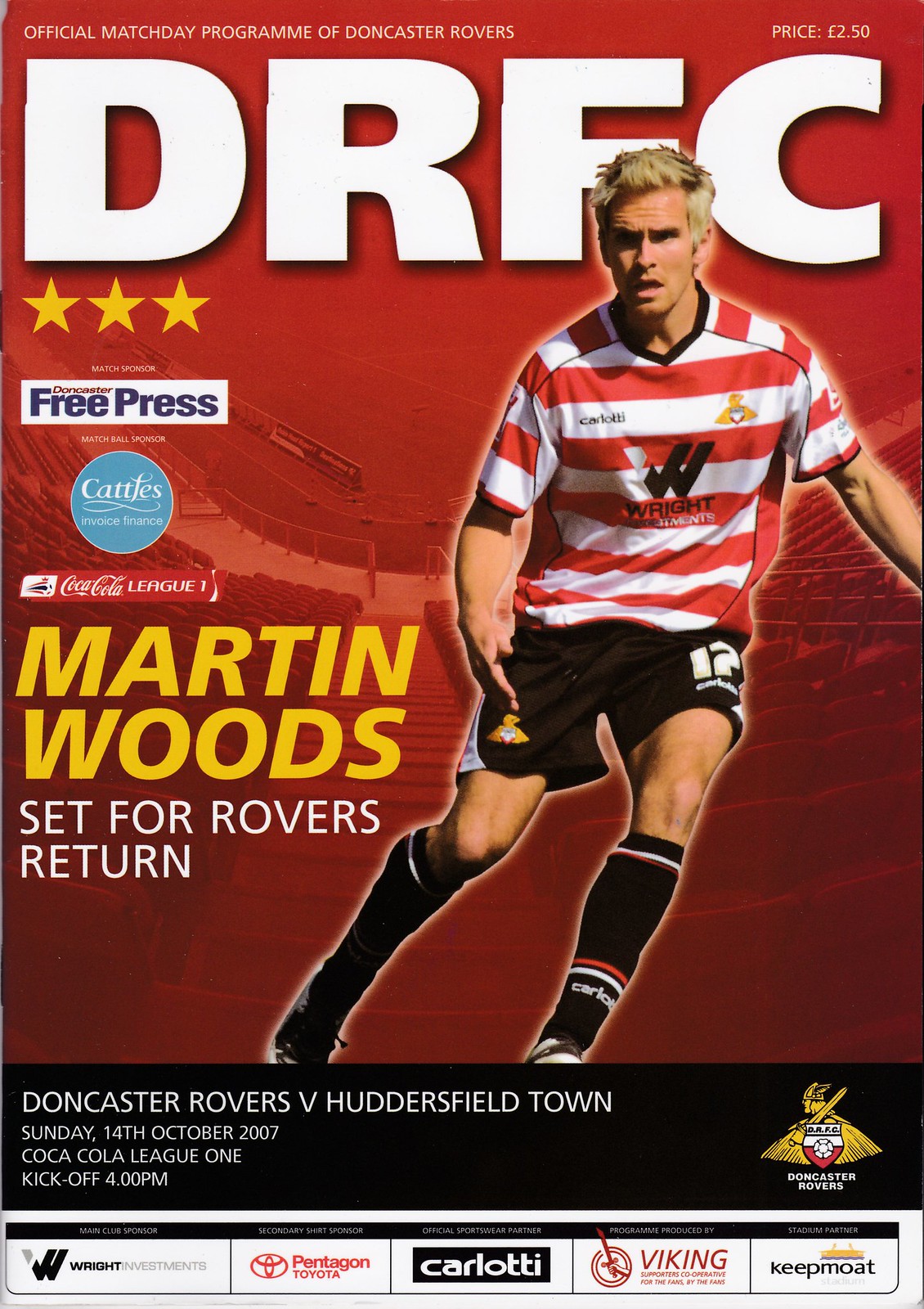This is the cover of an official match day program for Doncaster Rovers vs. Huddersfield Town on Sunday, October 14, 2007, with a kickoff at 4 p.m. The price of the program is £2.50, indicated at the upper right. Centered in large white letters are the initials "DRFC," standing for Doncaster Rovers Football Club. Below this, in a white rectangular box, is the text "Free Press," positioned to the center left. Adjacent to it, on the center right, is a photo of Martin Woods, dynamically captured in motion, leaning to the right in a horizontally striped white and orange jersey with black shorts. His name appears in bold yellow letters at the bottom, with the subtitle "Set for Rovers return" in white letters beneath it. A black banner with the Doncaster Rovers' club crest, predominantly red and gold, spans the bottom. Additional advertisements and the Coca-Cola League logo are situated towards the bottom of the cover.